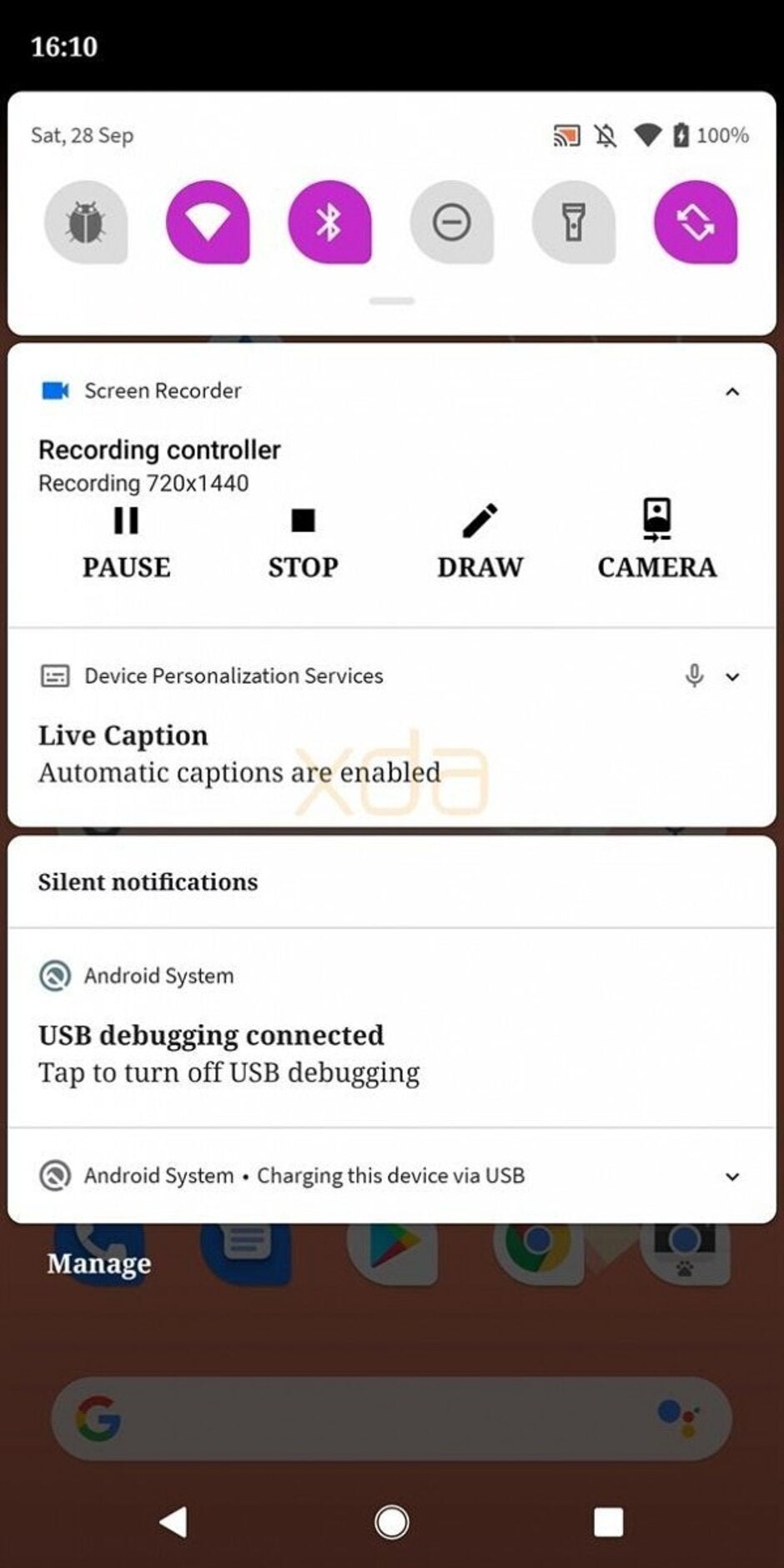Screenshot of a smartphone screen displaying essential status and utility information at 16:10 on Saturday, September 28th. The device shows full battery life (100%), connected to a Wi-Fi network, and no pending notifications. The top portion of the screen includes several icons in either gray or purple boxes, representing different functions: a bug icon (possibly for developer options or an error), Wi-Fi, Bluetooth, a circle with a line through it (perhaps signifying 'Do Not Disturb' mode), an icon resembling either a flashlight or a trash can, and an unidentified icon. 

Below these icons, the screen indicates 'Screen Recorder' is active, with an ongoing recording resolution of 720 x 1440. Control options such as 'Pause', 'Stop', 'Draw', and 'Camera' are listed. The device also displays 'Device Personalization Services', 'Live Caption' with 'Automatic Captioning Enabled', and a 'Silent Notification' about the 'Android System'. Additionally, there is a notification stating 'USB debugging connected' with an option to turn it off, and confirmation that the device is 'Charging via USB'.